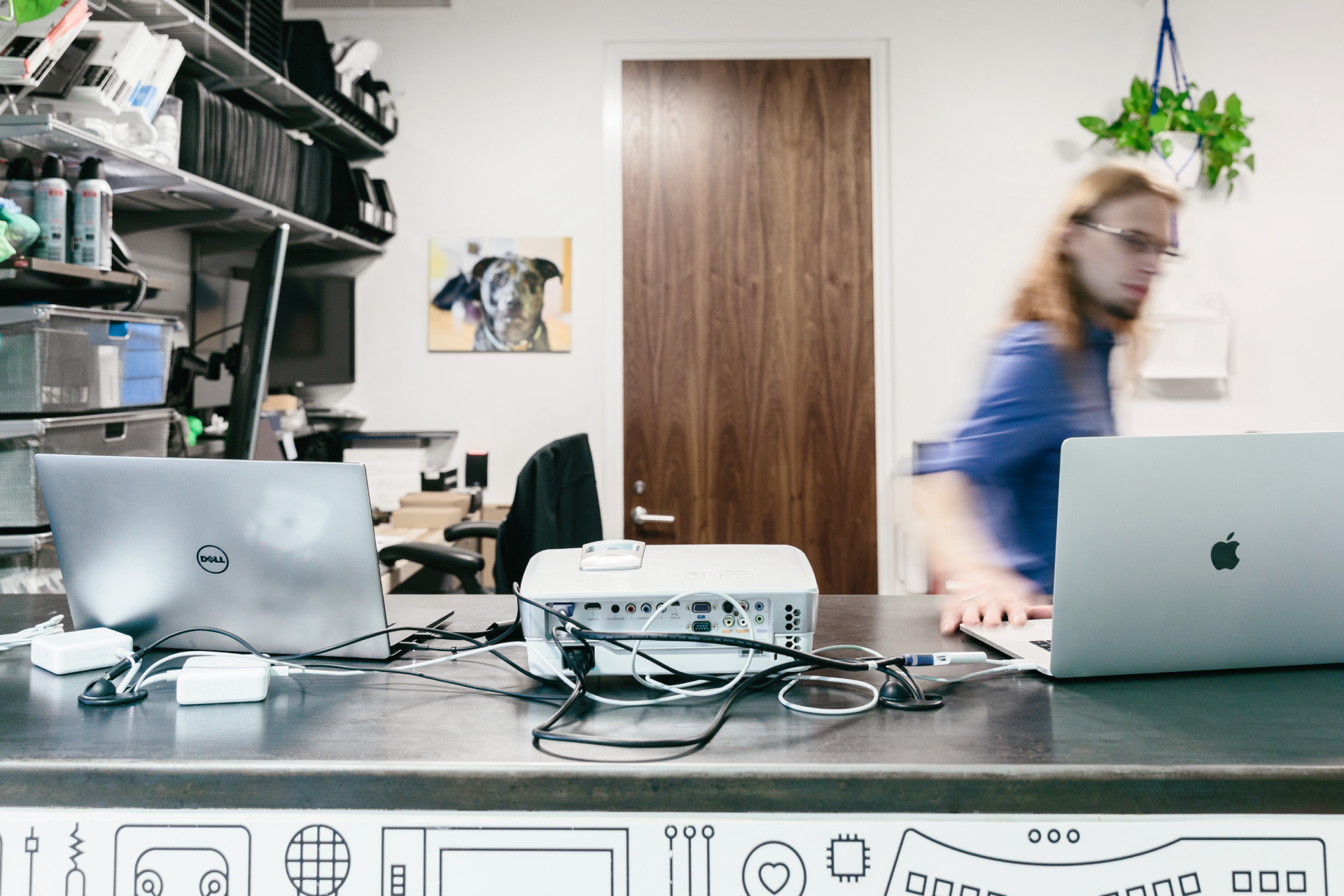The image showcases a busy scene inside what appears to be a computer store or repair shop. At the front counter, a man is seen operating two laptops— a silver Dell PC laptop on the left and a similarly silver or dark gray Apple MacBook on the right. Between the laptops, there is a central white hub connecting them both, presumably to the same network.

The man, who has long hair, glasses, and a thin beard or goatee, is captured in motion, his blurred form indicative of his active nature. His hand rests on the keyboard of the Apple laptop. He is wearing a blue shirt and is positioned behind the counter amidst a clutter of technical tools and accessories, including cans of compressed air for cleaning components, and plastic tubs filled with cords and various parts.

The background reveals a detailed interior; there's a brown wood grain door with a straight metal handle and a hanging pot. To the right of the frame, there's a painting of a dog on the wall, along with shelves and cabinets that store additional items. The countertop holding the laptops also features an electrical design at its base, complementing the tech-focused setting.